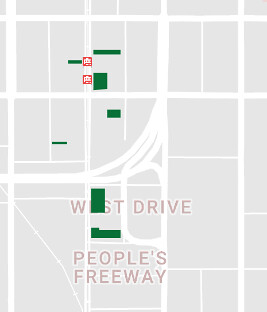Detail of a digital map, likely captured from a cell phone screen, displaying a section of a city. The background is a uniform pale gray, setting the stage for a labyrinth of white roads in grid and arched patterns, indicating both straight and curving streets. A broad highway interchange is prominently visible, arching through the center of the image and effectively dividing the map into quadrants.

Scattered across the map are mysterious green squares and rectangles in various shapes, the purpose of which is unclear. Additionally, two small, unreadable red boxes with white logos dot the map, possibly signifying landmarks or points of interest.

The top of the image is marked by a large label reading "West Drive," with a subtext of "People's Freeway" situated towards the bottom. This naming adds to the confusion as it’s not obvious what features these labels are referring to. The absence of direction arrows and street names, typically displayed in black font over the white roads, leaves the map difficult to decipher.

Overall, the image showcases a convoluted snippet of a larger city map, hampered by obscure labels and missing details that might become clearer upon zooming in.